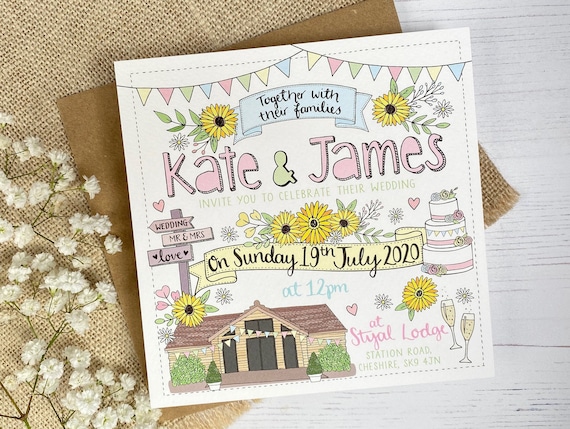The invitation is displayed on a background featuring a white-painted wooden surface and a sackcloth material above it. The invitation itself is a colorful, square-shaped card with a black dashed border. It boasts hand-drawn illustrations of delicate white flowers on thin stems, multicolored flag streamers, and a variety of quaint graphics. At the top, the names "Kate and James" are prominently written in a large, pink hand-drawn typeface with a green ampersand in between, shaded with pen lines for a whimsical effect. Surrounding the names are yellow flowers and a light blue ribbon banner with cursive text reading "together with their families."

Beneath the main header, light green text invites guests to celebrate their wedding. A smaller yellow banner underneath specifies the date, "on Sunday, 19th July 2020." Additional charming illustrations enrich the invitation, including a three-tiered cake, a signpost reading "wedding Mr. and Mrs. Love" with designs of a church or house, and champagne flutes, signifying a joyous celebration. The event details conclude with the venue information, "Styal Lodge, Station Road, Cheshire, SK9 4JN." This invitation is both detailed and festive, perfectly encapsulating the joyous occasion it heralds.